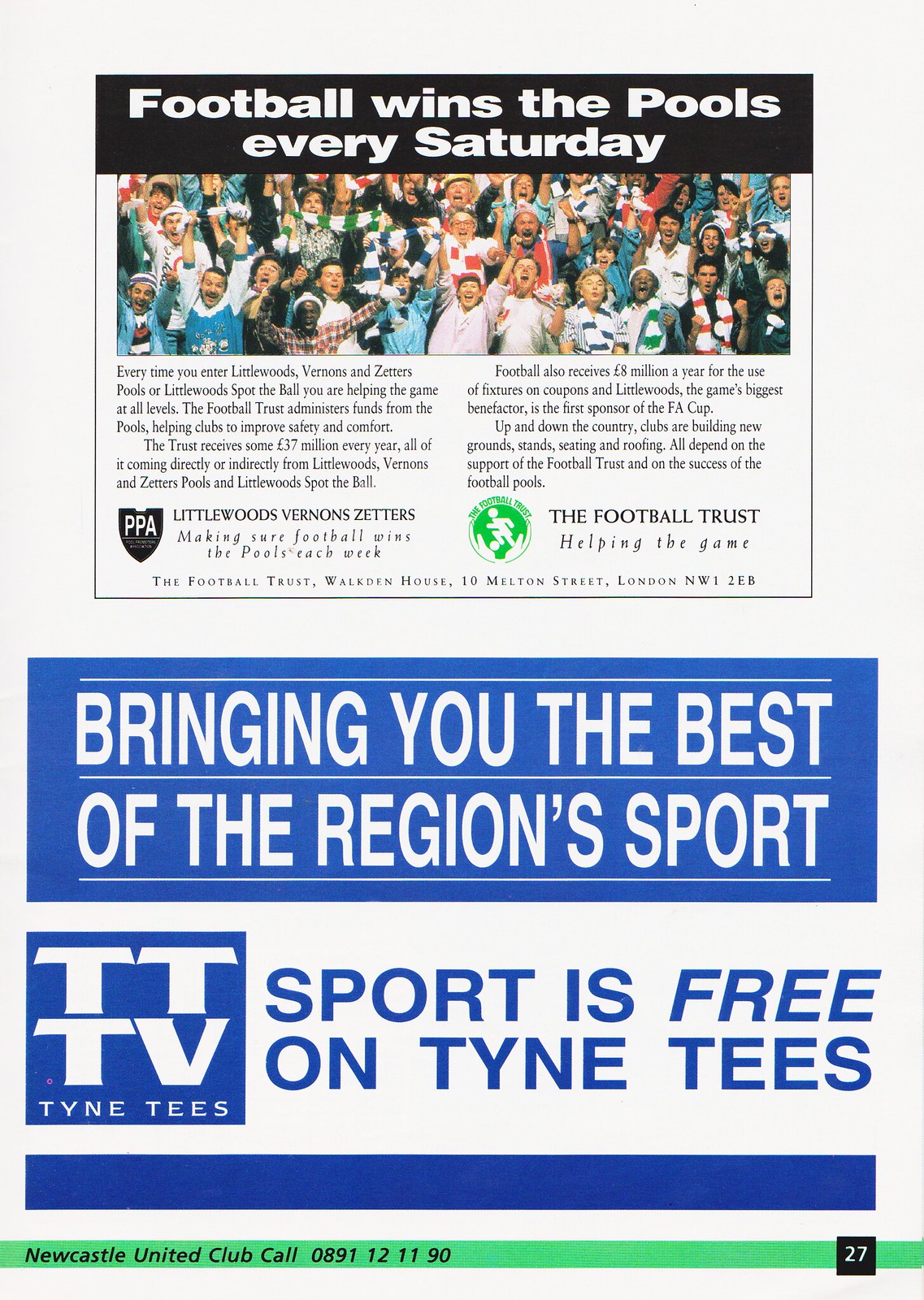This image appears to be a magazine or newspaper ad with a predominantly white background and accenting squares and banners. At the top, there's a black banner with white text stating, "Football wins the pools every Saturday." Below this banner is a vivid picture of a jubilant crowd, clad in variously colored shirts such as red, blue, and white, with many spectators raising their fists in celebration and cheering for their team.

Under the picture, there are paragraphs of text with phrases like "Littlewoods Vernon Zetters making sure football wins the pools each week" and "The Football Trust helping the game." Towards the bottom portion of the ad, a large blue banner with bold white text proclaims "Bringing you the best of the region's sport." To the left of this banner, there is a blue logo for "Tyne Tees" and to the right, in blue text, it says, "Sport is free on Tyne Tees."

Beneath these elements, a green banner features black text that reads, "Newcastle United Club Call 0891-121190." Finally, the page is marked with the number "27" inside a black square located at the bottom right corner, indicating perhaps the page number or some form of categorization.